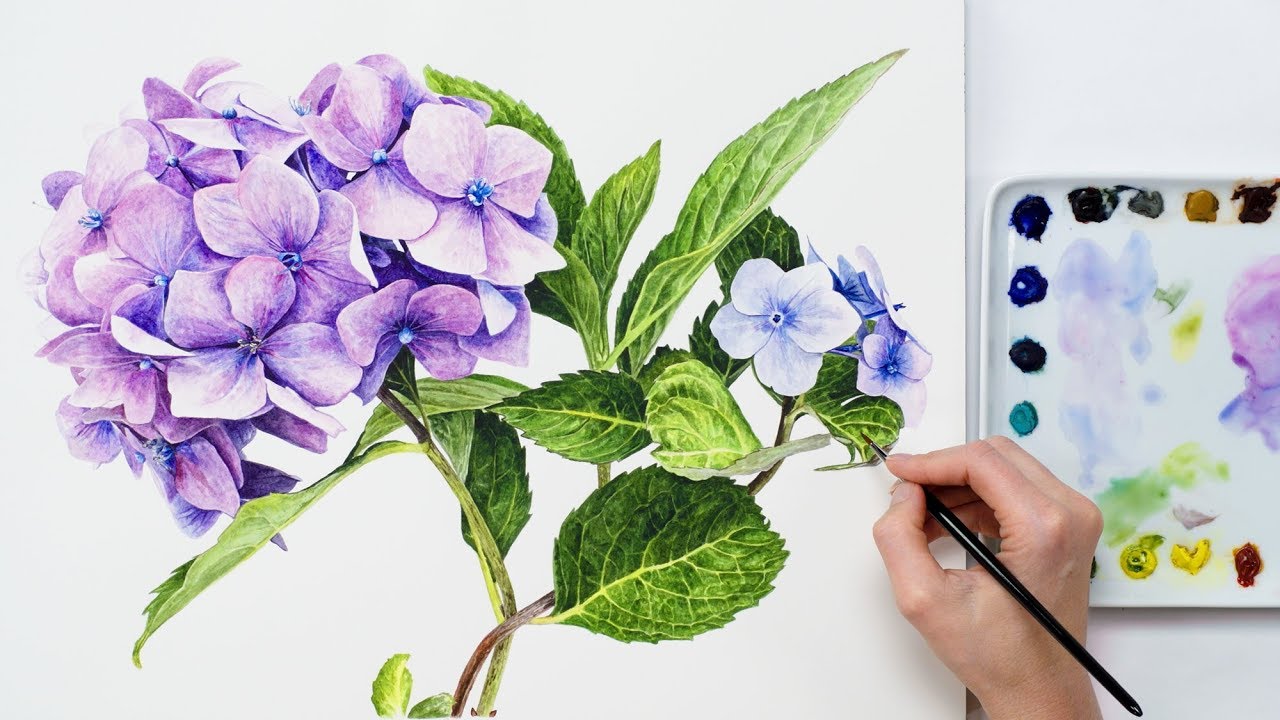Overhead shot of a watercolor painting in progress, showcasing only the artist's right hand holding a skinny, black watercolor paintbrush. The painting features a large cluster of detailed purple flowers on the left side, with vibrant green leaves and stems dominating the right side. On the extreme right, two small blue flowers with delicate petals contrast with the larger purple blooms. Adjacent to the hand, a white palette bursts with a variety of colors—blacks, blues, greens, yellows, pinks, oranges, and reds, some of which are blended. The scene captures the dynamic process of creating art, set against a white work surface.